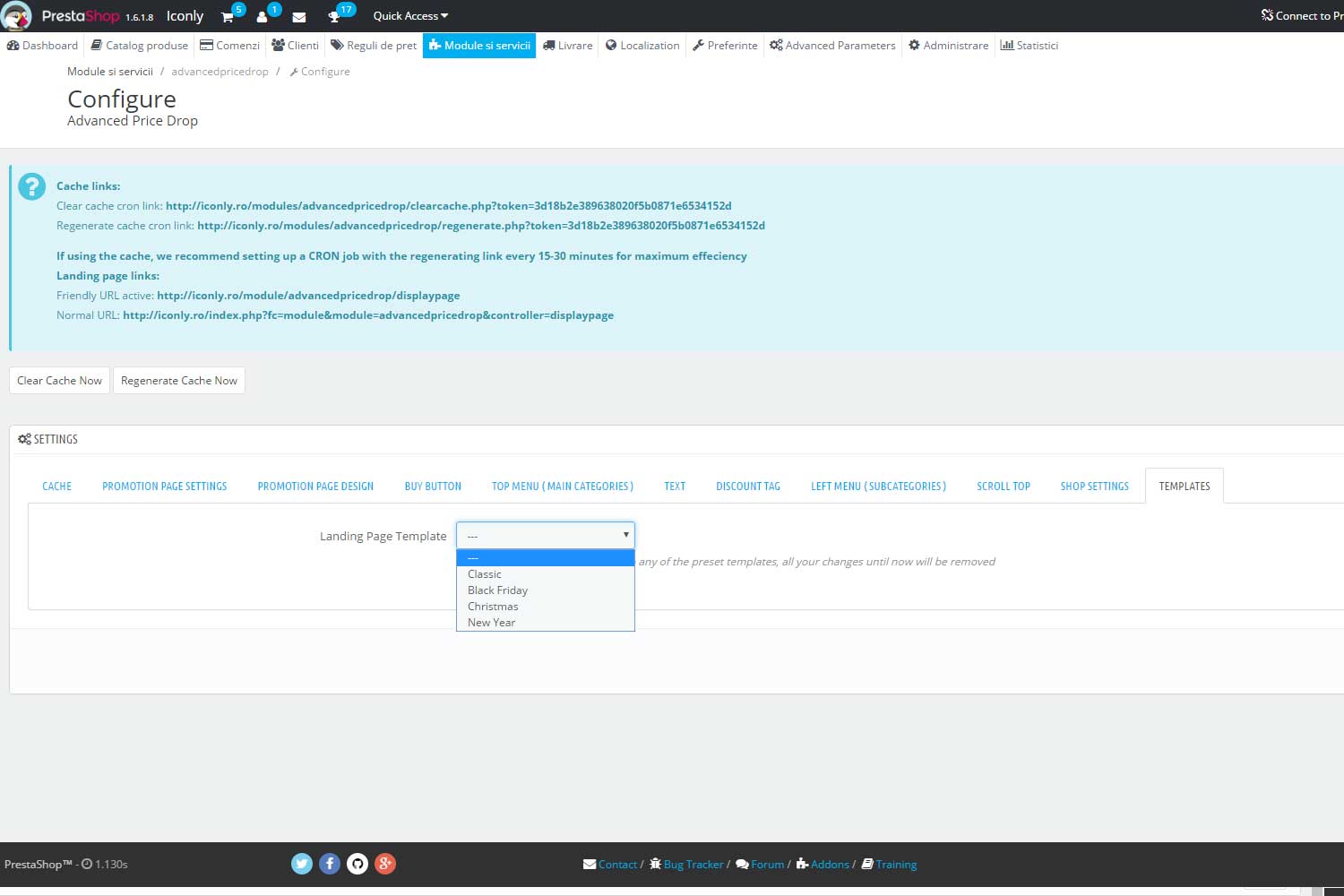The image depicts a website interface likely associated with PrestaShop, an e-commerce platform. The header prominently features the word "Presta" in white letters followed by "shop" in pink. Next to this branding, there's an icon of a shopping cart, though the number of items within it is too small to discern clearly. Adjacent to the cart is a profile icon, potentially indicating one notification or user detail at the top. There is also an envelope icon and another symbol resembling a reward, which displays the number 17.

On the left sidebar, the navigation menu includes options for:

1. Quick Access
2. Dashboard
3. Catalog - part of the word is obscured
4. Clients - partially cut off
5. A section possibly in another language
6. Modules
7. Another entry beginning with an 'S'
8. Another entry beginning with an 'L' – maybe 'Localization'
9. An entry starting with 'P'
10. Advanced Parameters
11. Another section with 'A' 
12. Statistics

At the bottom of the sidebar, there's a "Settings" section. Additionally, there's a dropdown menu with various templates for different occasions – "Landing Page," "Classic," "Black Friday," "Christmas," and "New Year."